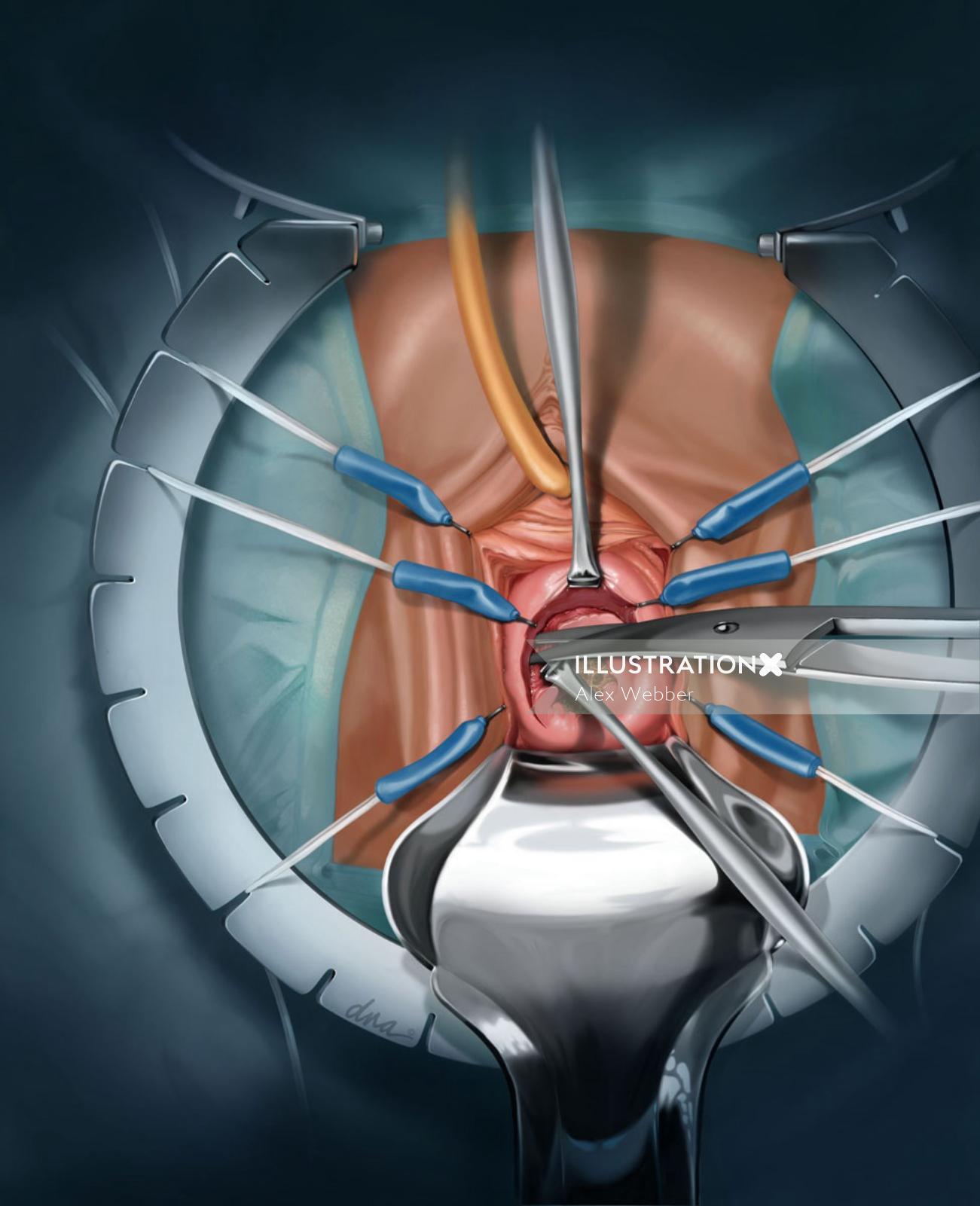This detailed medical illustration by Alex Weber vividly depicts an abdominal surgical procedure. The focal point is a round metal frame positioned over the patient's partially exposed abdomen, which is otherwise covered with blue surgical drapes. The open area reveals an incision, wide open with the assistance of hooks attached to rods on the metal frame and metal forceps at the bottom. These tools ensure a clear view of the internal structures, including a visible pinkish round structure within the incision. Inside, there is also a metal rod and possibly a robotic arm navigating a yellow tube extending into the body. The entire scene suggests an intricately managed surgical environment, showcasing various instruments meticulously holding and accessing the internal tissue. The digital nature of the artwork is affirmed by a watermark that reads "Illustration by Alex Weber."